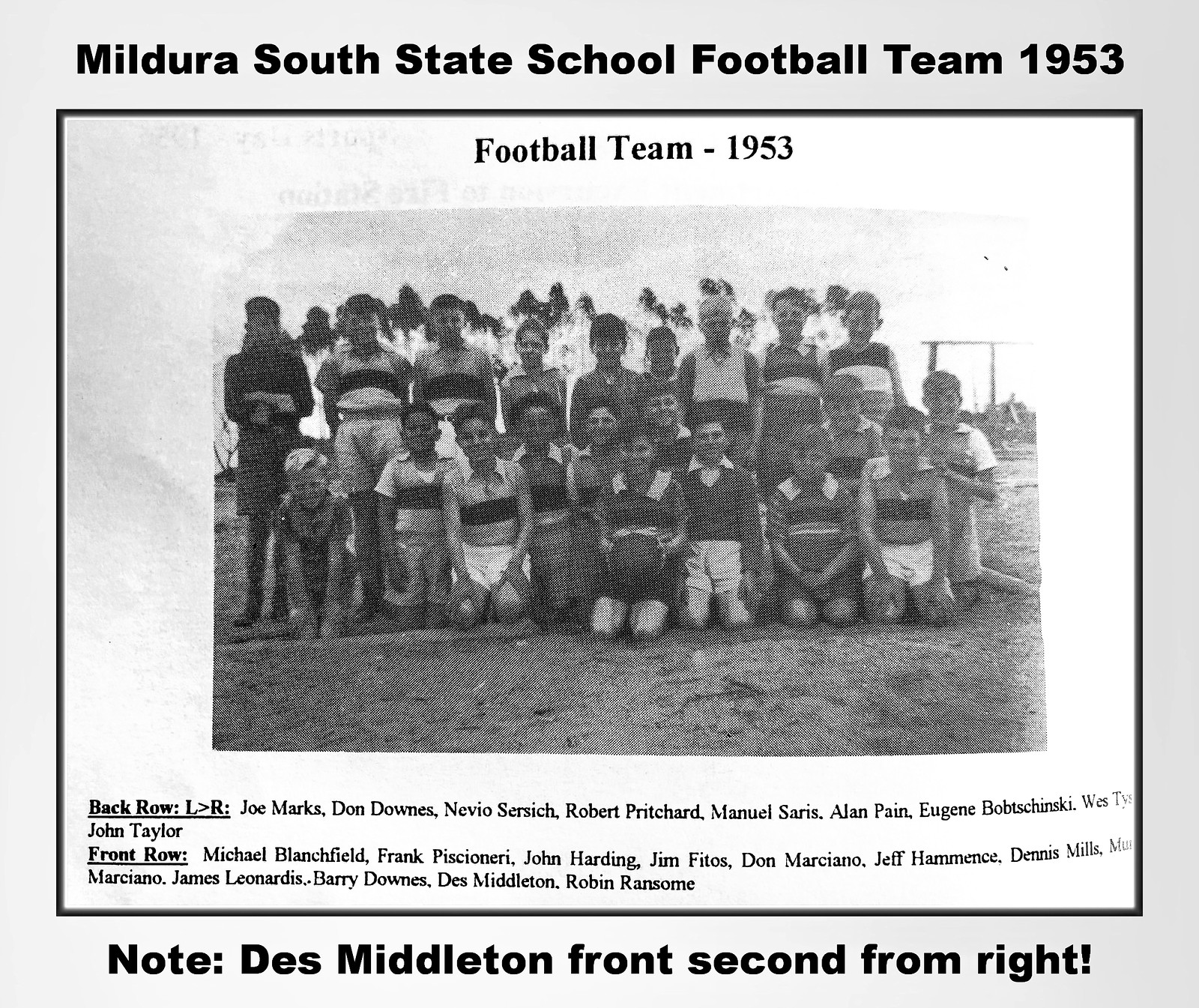The rectangular photograph, framed with a white border and a black trim, depicts the "Mildura South State School Football Team, 1953." This title appears prominently at the top and again just above the photo itself. The black-and-white image, of somewhat poor quality with a thatched appearance as if printed by a low-quality dot matrix printer, shows a youth football team. The children, approximately 9 to 11 years old, are arranged in two rows with additional kids kneeling to form a partial third row. Despite some damage to the top corners, the team members can still be discerned. Beneath the photo, there are listings for the back row and front row, denoted as "Back Row (left to right)" and "Front Row (left to right)," respectively, which provide the names of each player. The names include Joe, Don, Nevio, Robert, Manuel, Alan, Eugene, Wes, John, Michael, Frank, John, Jim, Don, Jeff, Dennis, James, Barry, Des, and Robin. Notably, there is a specific mention: "Des Middleton, front second from right." This detailed labeling serves as a legend to identify and point out each player in the photograph.